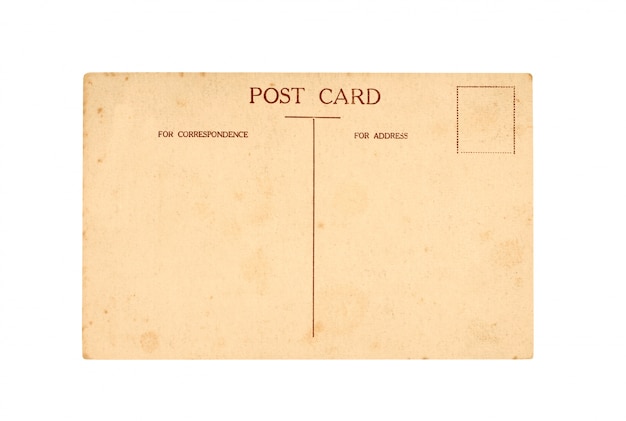This image depicts a very old and aged postcard, distinguished by its brownish-tan color, likely a result of its several years of age, although it may have once been white or pale yellow. The postcard is blank, devoid of any personal content or address. At the top, "POSTCARD" is prominently displayed in large, dark letters. Below this title, there is a small horizontal line intersected by a long vertical line in the center, forming a T-shape. On the left side of the vertical line, it is labeled "FOR CORRESPONDENCE," while the right side reads "FOR ADDRESS." Additionally, there is a small rectangular box in the upper right-hand corner designated for a stamp. The overall appearance of the postcard, with its light brown smudges and faded text, accentuates its vintage quality.